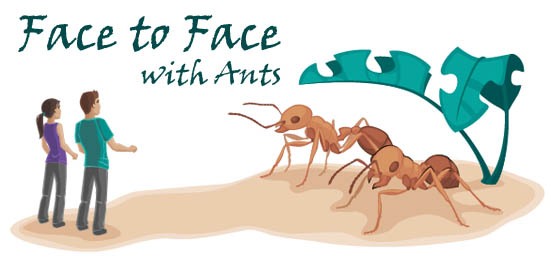This hand-painted-style graphic illustration, titled "Face to Face with Ants" in a bluish-green handwritten font at the top left, features two people and two gigantic ants against a white background. The surreal scene places the two figures, a teenage boy and girl, in the left center. They appear shocked, with arms outstretched and backs arched. The girl, with brown hair tied back in a ponytail, wears a purple shirt and gray pants, while the boy, with short brown hair, sports a teal shirt and gray pants. Opposite them on the right, the two enormous ants, larger and longer than the humans, dominate the scene. Behind the ants, two green leaves resembling umbrellas add a naturalistic touch. The entirety sits atop a small patch of land, suggesting a fantasy book or story illustration.